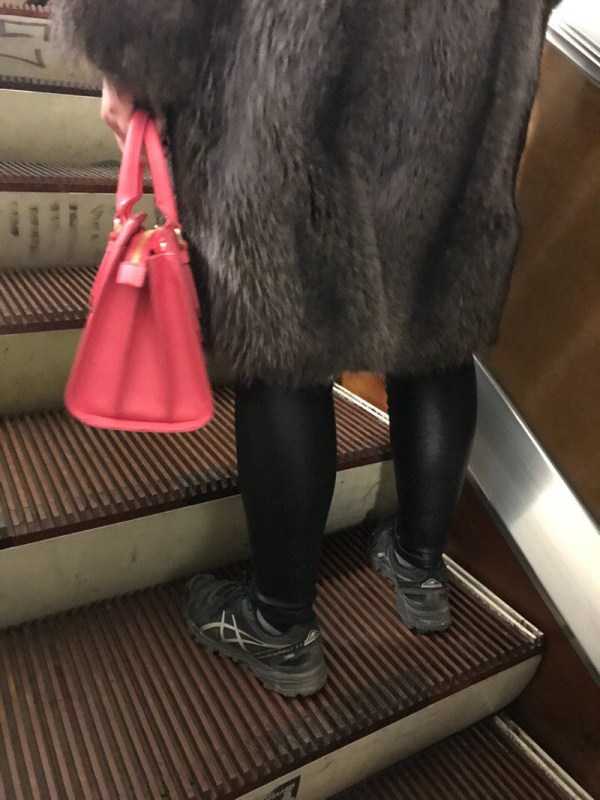A woman is captured from the backside, waist down, standing on an ascending escalator. She wears black leggings that have a sheen, resembling leather, paired with a dark gray, knee-length fur coat. Her footwear includes black sneakers featuring a silver wave design on the side. In her left hand, she holds a trapezoid-style pink leather handbag with matching handles. The escalator steps are dark brown with a lighter brown outline along the ridges, and the sidewall of the escalator is a coffee brown color with a silver strip acting as a border where the molding would be. The image focuses on the details from her hips down, highlighting the textures and colors of her outfit against the background of the escalator.